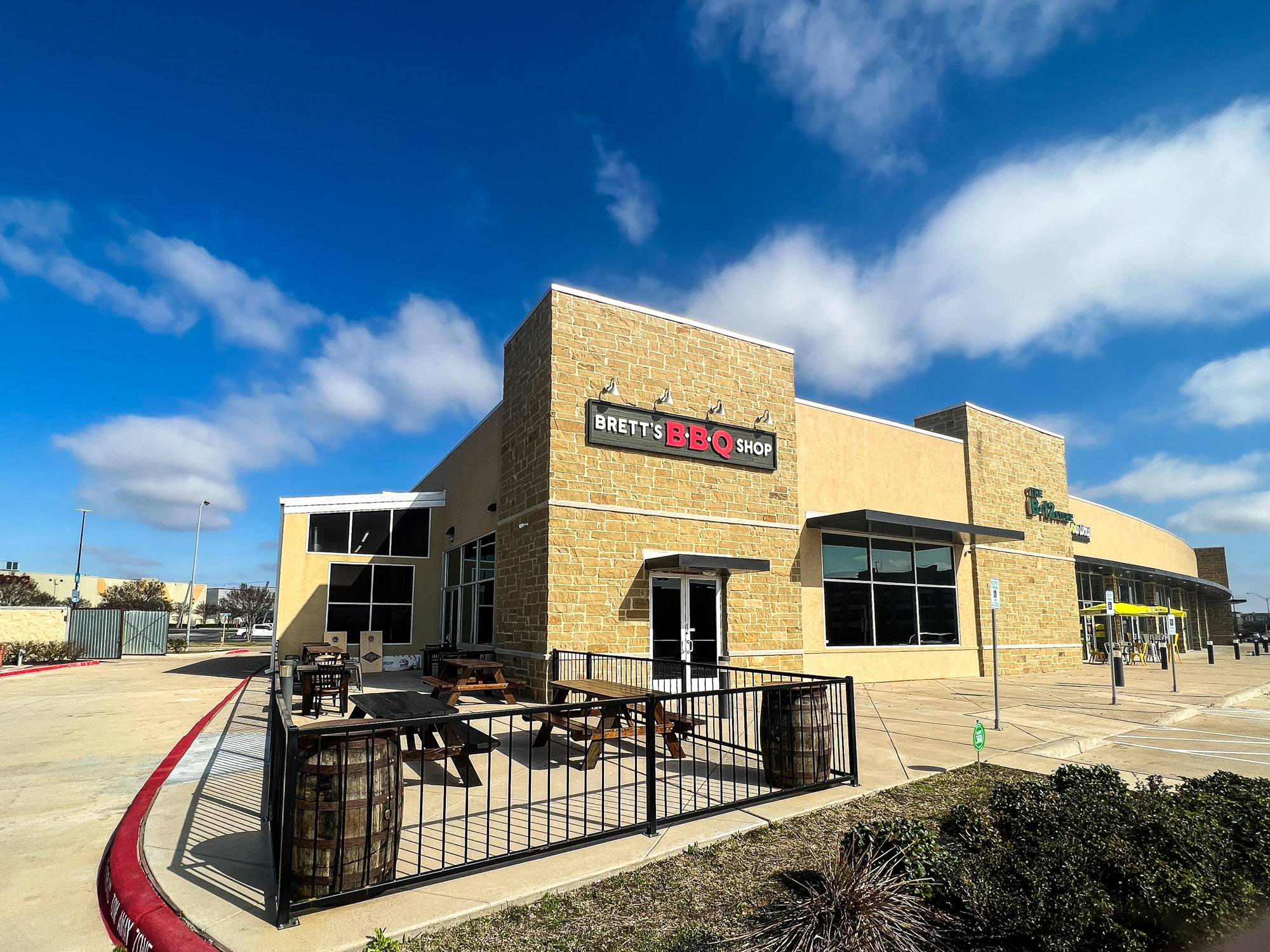This is a rectangular, landscape-oriented photograph taken outdoors during the daytime, capturing the front view of a strip mall under a blue sky dotted with fluffy white clouds. The sky transitions from a lighter blue at the horizon to a darker shade towards the top left. The main building featured is a yellowish-tan, stone-patterned structure that extends from the right almost to the lower left corner of the image. A prominent corner store, Brett's BBQ Shop, commands the center of attention with its black rectangular sign bearing bold white letters for "Brett's," larger red letters for "Barbecue," and "Shop" again in white. This sign is illuminated by lights above. Below the sign and to the left of the entrance, there's a patio area enclosed by black iron fencing, furnished with picnic tables and some old wooden barrels, adding to the rustic charm. The building boasts a brick design, and the doorway has a distinctive white border. To the right, parking signs are visible, and part of the curb is painted red, indicating a driveway or throughway in front of the building. Some bushes can be seen at the bottom right corner of the image, adding a touch of greenery to the overall scene.